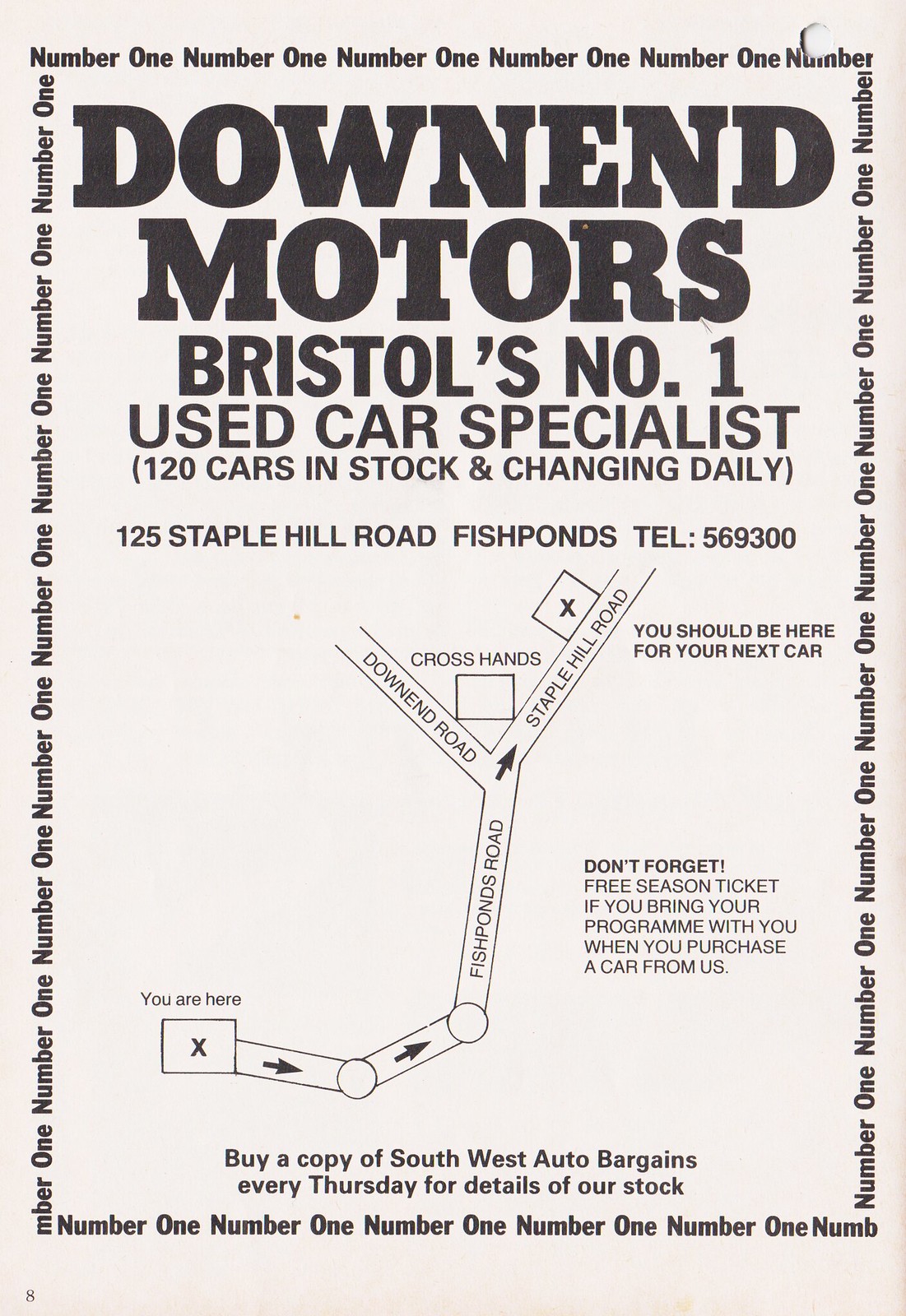This vertical, rectangular advertisement, likely from a newspaper or magazine, features a classic gray background with black text. The entire frame is bordered by a continuous repetition of the words "number one." At the top, in large, bold, uppercase letters, it proclaims "DOWN END MOTORS." Directly underneath, "Bristol's number one used car specialist" is noted in slightly smaller font. Further, it mentions, "120 cars in stock and changing daily," followed by the dealership's address, "125 Staple Hill Road, Fish Ponds," and the telephone number, "569-300."

Dominating the advertisement's lower half is a detailed, stylized map directing potential customers to the dealership. The map starts with an "X" labeled "you are here" and includes arrows showing the route along Fish Ponds Road, which forks into Staple Hill Road on the left and Downs End Road on the right. An intersection landmark, identified as 'Crosshands,' is centrally placed within this junction. Next to a square on Staple Hill Road, the text reads, "You should be here for your next car."

Beneath the map, a reminder tells customers, "Don't forget free season ticket if you bring your program with you when you purchase a car from us." At the very bottom, in smaller print, it advises, "Buy a copy of Southwest Auto Bargains every Thursday for details of our stock."